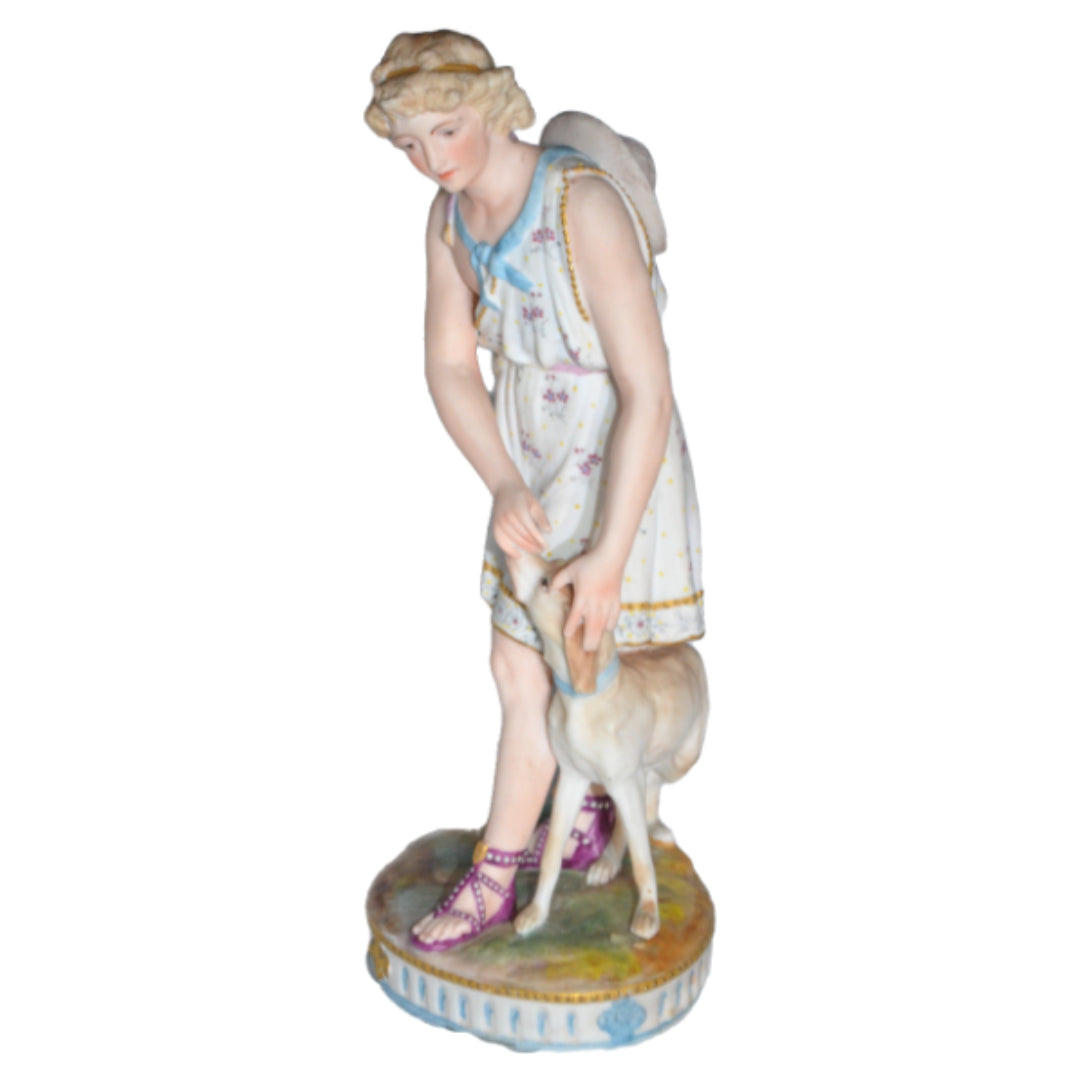This image showcases a detailed, porcelain-like figurine of a little girl and her dog, both carefully positioned on a small ceramic pedestal. The pedestal features a light blue base with darker blue vertical stripes and a prominent blue diamond at its front, while the top is painted in earthy tones of green, orange, and yellow, resembling natural ground. The girl has short blonde hair and wears a white dress adorned with pink floral patterns and a blue neckline. Her dress reaches down to her knees, revealing her purple high-heeled sandals. Notably, she has a hat secured around her back, hanging by her neck. She is bent over, reaching down with both hands to pet her dog, who nestles partly under and behind her dress. The dog, a small hound-like breed, is white with light brown patches and looks up affectionately as she pats its head and rubs its nose. Both the girl and the dog exhibit a tender, innocent expression, capturing a moment of shared affection.